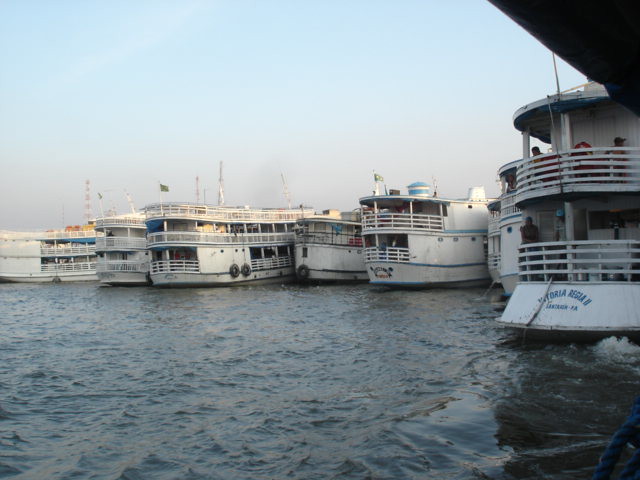This outdoor image features a line of six large passenger ships, possibly yachts or dinner cruise ships, docked in a body of water. The water appears slightly rough, suggesting movement. Each ship is equipped with two or three decks, where people can be seen standing or sitting, enjoying the view. The sky above transitions from a clear blue at the top to a more cloudy, whitish hue at the horizon, adding depth to the scene. In the upper right-hand corner, there is a black triangular shape, likely the roof of a nearby structure. The boats have writing on them, some in blue and others in blue and yellow, though the text is too small to discern. Overall, the photo captures a serene yet lively snapshot of these large vessels and their surroundings.